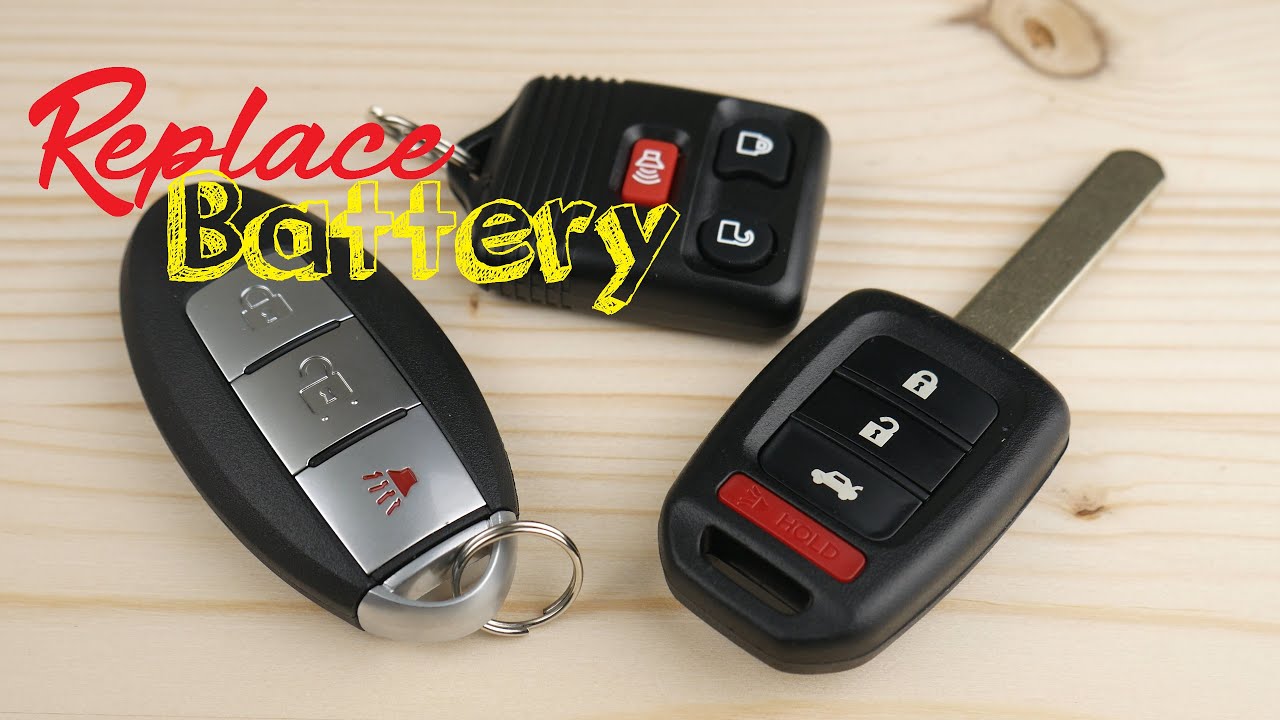The image displays three different black electronic vehicle fobs on a lightly colored, untreated wooden surface. At the top of the image, overlayed text reads "Replace battery" in red cursive, with "battery" highlighted in yellow and given a 3D shadow effect.
 
On the left, a predominantly black oval-shaped fob features three silver buttons: a lock button, an unlock button, and a honk button with a red symbol resembling a speaker. It also includes a keychain ring. 

The central fob has a simpler design, with two buttons for locking and unlocking, and a red button in the middle that likely acts as another honk function. This fob also includes a key ring.

On the right, a more complex square-shaped fob includes three buttons, each marked with icons for lock, unlock, and trunk release. It features a distinctive silver protrusion that resembles a popsicle stick and a red bar at the bottom. 

These fobs are placed on a light brown wooden surface that appears untreated, with visible rings and texture adding to the image's rustic feel.